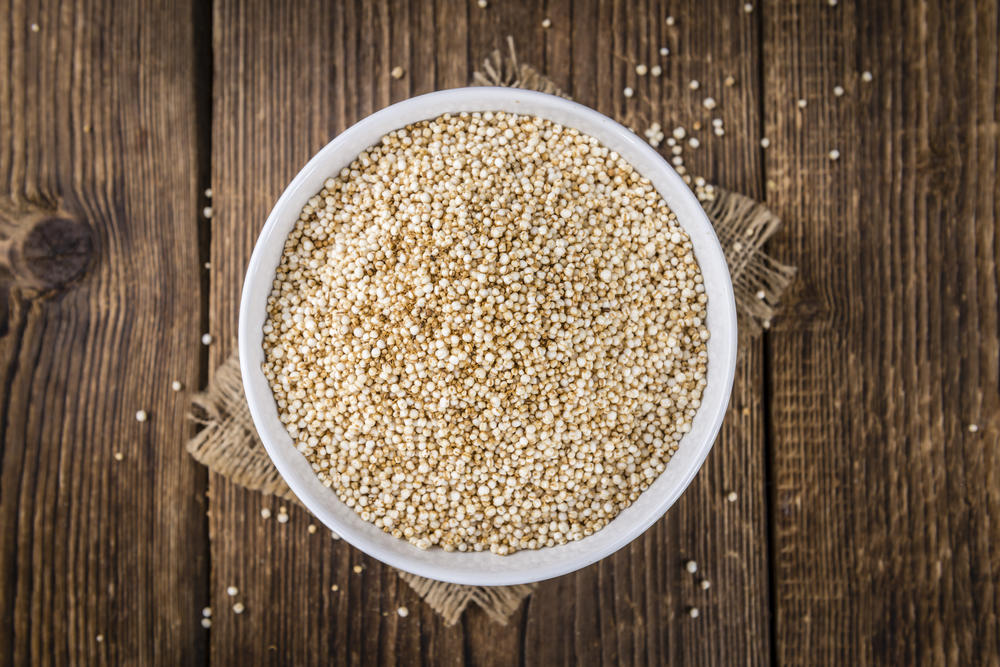This detailed photograph captures a white bowl filled to the brim with a tan-colored grain, possibly quinoa or a similar small seed, each grain being less than a millimeter in size. The white bowl sits at the center of the image, resting on a burlap cloth, which acts as a rustic placemat atop a dark-stained wooden table. The table features three vertical, distressed planks with a shabby chic aesthetic, including a noticeable knot on the left side. Some grains are scattered around the bowl, onto the burlap and wooden surface, enhancing the naturalistic and casual setting. The lighting is of professional quality, suggesting a commercial or high-end photographic context.